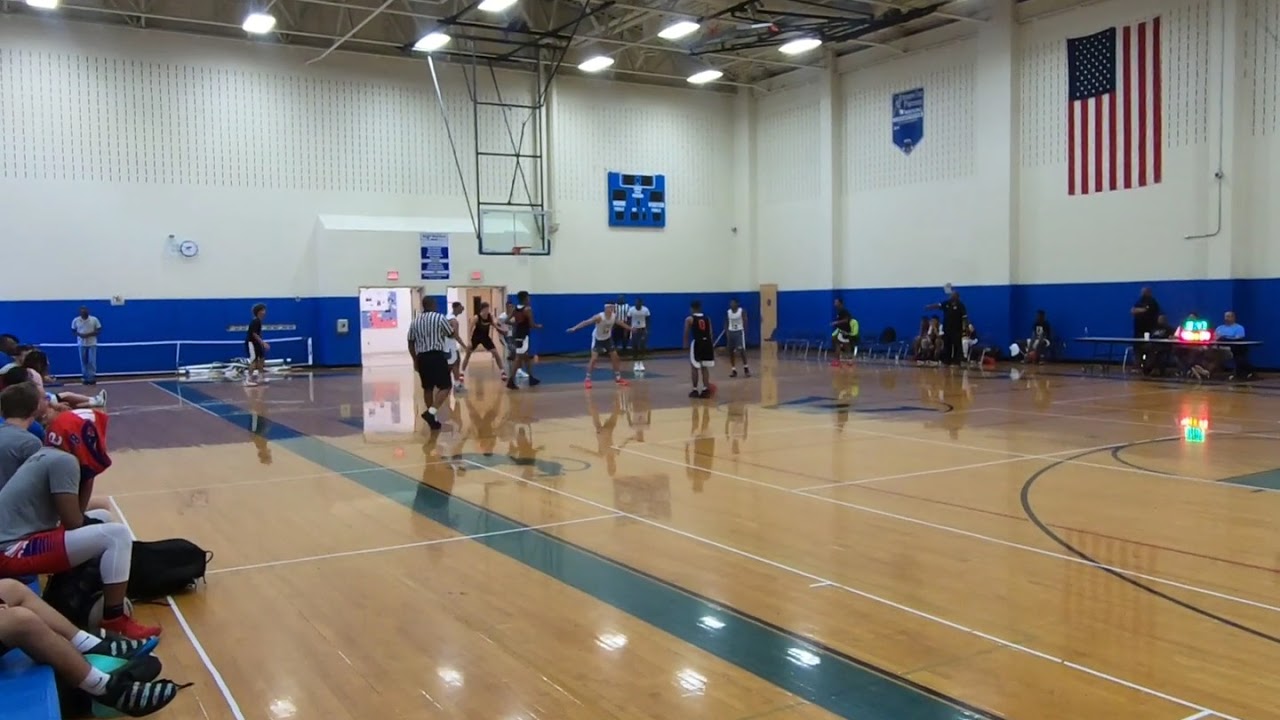The image depicts a lively basketball game taking place inside a school gymnasium with shiny wooden floors. On the court, one can see two teams: one adorned in black, red, and white uniforms, and the other in white jerseys paired with blue shorts. The game is being closely watched by a referee wearing a black and white striped shirt and black shorts. The gymnasium features white walls accented with blue padding typical of school gyms. Above, a retractable glass backboard is in use, while a blue scoreboard and banners adorn the walls, though the scoreboard is not currently active. An American flag hangs upside down, positioned near a score table to the right of the scene, which features an LED scoreboard and is surrounded by some seated and standing spectators. Blue bleachers line one side where additional viewers are seated. The ceiling lights reflect off the polished floor, and several open doors are visible in the background.